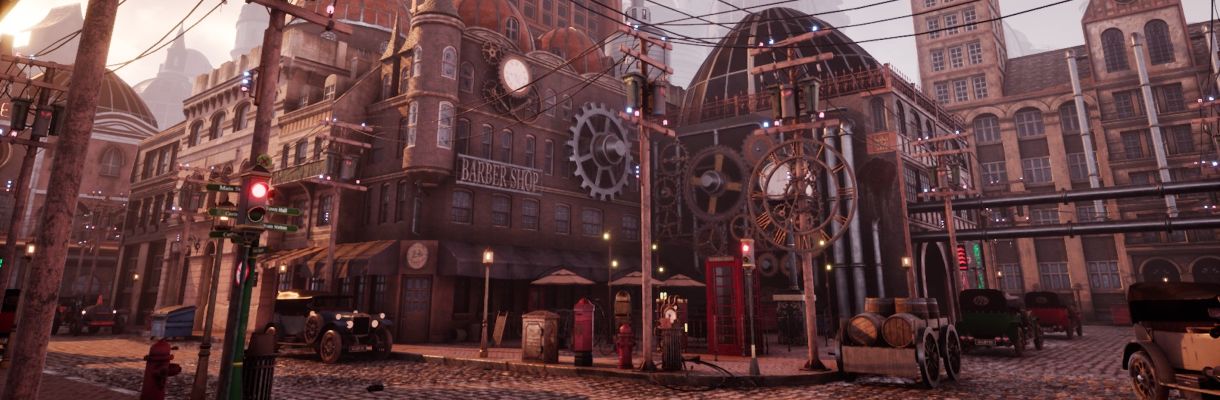The image is a detailed screenshot from a video game environment depicting a retro-futuristic city street corner reminiscent of the 1920s or 1930s. The scene showcases a mix of old-style architecture and advanced mechanical elements. Dominating the left side is a large brown brick building with a prominent "Barbershop" sign and an attached metal gear, adding to the vintage ambiance. In front of this building is an empty street bordered by a traffic light, currently red. Close to the sidewalk, a black car and a blue dumpster can be seen, suggesting urban activity. On the right side of the street, there is another building also adorned with gears, and standing at the edge of the sidewalk is a pole featuring clock symbols. The right side of the scene includes a carriage filled with barrels, contributing to the historical feel. Additionally, electrical cables stretch between poles and buildings, integrating a subtle futuristic twist into this otherwise period-specific setting.